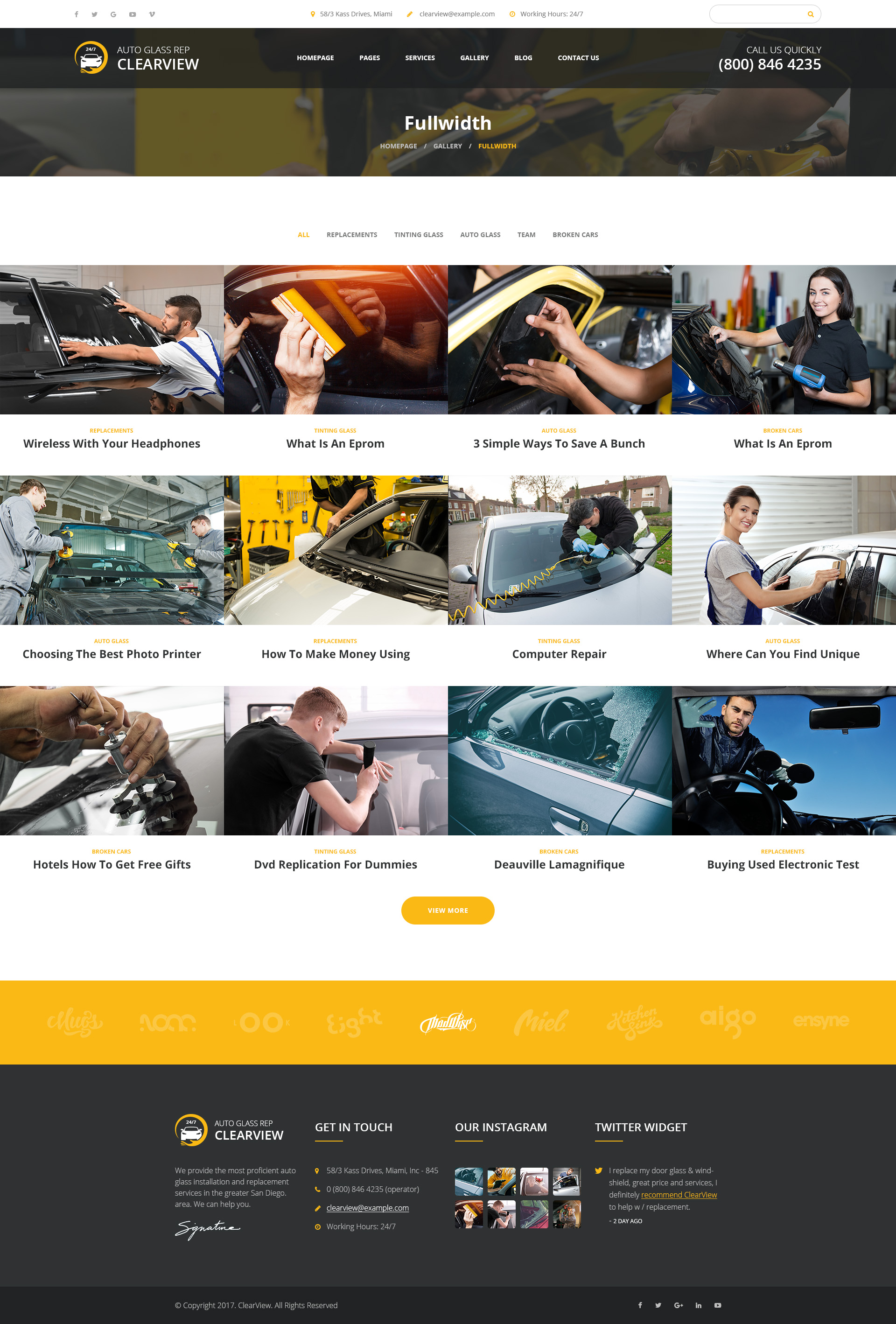This image is a screen capture from a website titled "Auto Glass Rep Clear View." At the top of the website, a menu bar provides various navigation options, though the text is somewhat small and difficult to read. To the right of the menu bar, there is a search box identified by a gold or yellow magnifying glass icon. Just below this, "Auto Glass Rep Clear View" is prominently displayed in white lettering on a black background, accompanied by a white car icon encircled in gold.

The navigation bar beneath the title offers a series of options that appear to include "Homepage," "Services," "Gallery," and "Contact." There is also a prominent call-to-action message stating, "Call us today, 800-846-4235," urging visitors to get in touch. 

The section following the navigation bar features the words "Full Width," suggesting a layout template, accompanied by various clickable options that likely lead to videos. Some of the video titles include "Wireless with Your Headphones," "What is an EPROM," "Three Simple Ways to Save a Bunch," "Choosing the Best Photo Printer," "How to Make Money Using Computer Repair," "Where You Can Find Unique Hotels," "How to Get Free Gifts," "DVD Replication for Dummies," "Beauville Magnifique," and "Buying Used Electronic Test Equipment." These are represented with associated icons, predominantly depicting auto glass installation themes and processes.

The next section seems to highlight various features or recognitions the company has received, set against a yellow background. Lastly, the website's footer contains a sitemap on a dark gray background with white lettering, offering additional navigation and organizational information.